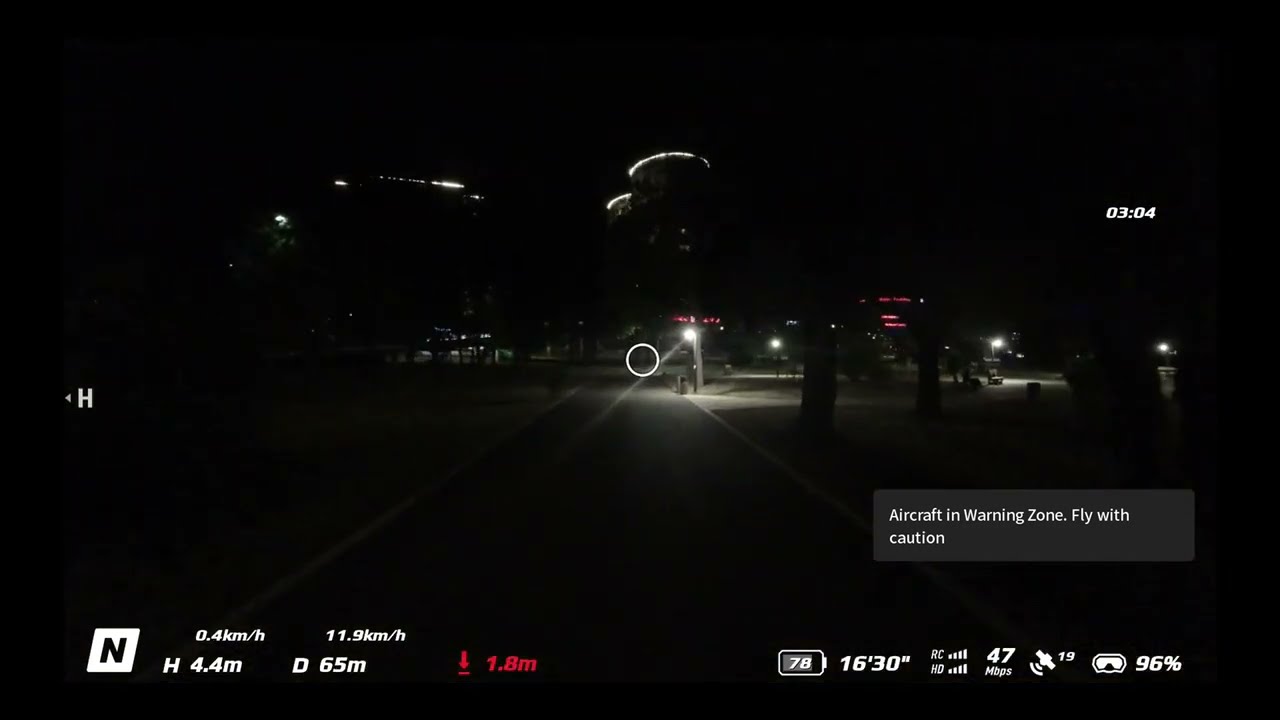The image is a dark, difficult-to-discern color illustration likely from a video game or flight simulator app, viewed in landscape orientation. Situated in what appears to be an outdoor setting, possibly a tarmac, the focal point is a dim light in the middle with indistinct lines suggesting a structure or football field-like layout. In the foreground, game stats and indicators are visible from a cockpit vantage point at night. A person is visible ahead, possibly guiding an aircraft with a flashlight. Detailed data is dispersed across the screen: on the lower right, a box reads "Aircraft in warning zone. Fly with caution," followed by statistics such as a battery percentage indicator showing "78", distances of "16 feet" and "30 inches", a wireless indicator at "47 Mbps," and various measures like "0.4 km/h" and "11.9 km/h". Next to an icon, perhaps ski goggles, lingers a number "96", with the letters "R", "C", and "H", followed by bars indicating progress. Additionally, the top right corner features a digital white clock, enhancing the gaming interface's immersive feel.